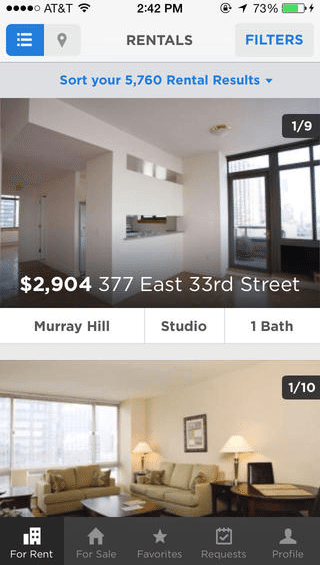This mobile screen capture shows a detailed view of a rental browsing app or website, with AT&T as the phone service provider and a connected Wi-Fi network. The current time is 2:42 p.m., displayed prominently at the top center of the screen. Standard icons such as orientation lock and location sharing are visible. The battery is at 73% and is currently charging.

The interface features a gray background with dark gray text and blue accent colors. A menu and pin marker button are located prominently. The central text reads "rentals," accompanied by a filter button. The screen also indicates that there are 5,760 rental results available for sorting.

Two property listings are partially visible on this screen. For the first listing, the rental price is $2,904 for a property located at 377 East 33rd Street in the Murray Hill neighborhood. This is a studio apartment with one bathroom. 

The screen shows an image carousel, with the first image depicting an empty entryway and labeled as one of nine images. The second image, labeled one of ten, features a staged living room with a fully set-up couch. 

At the bottom of the screen, there are navigation buttons labeled "For Rent," "For Sale," "Favorites," "Requests," and "Profile," allowing for easy user interaction and browsing.